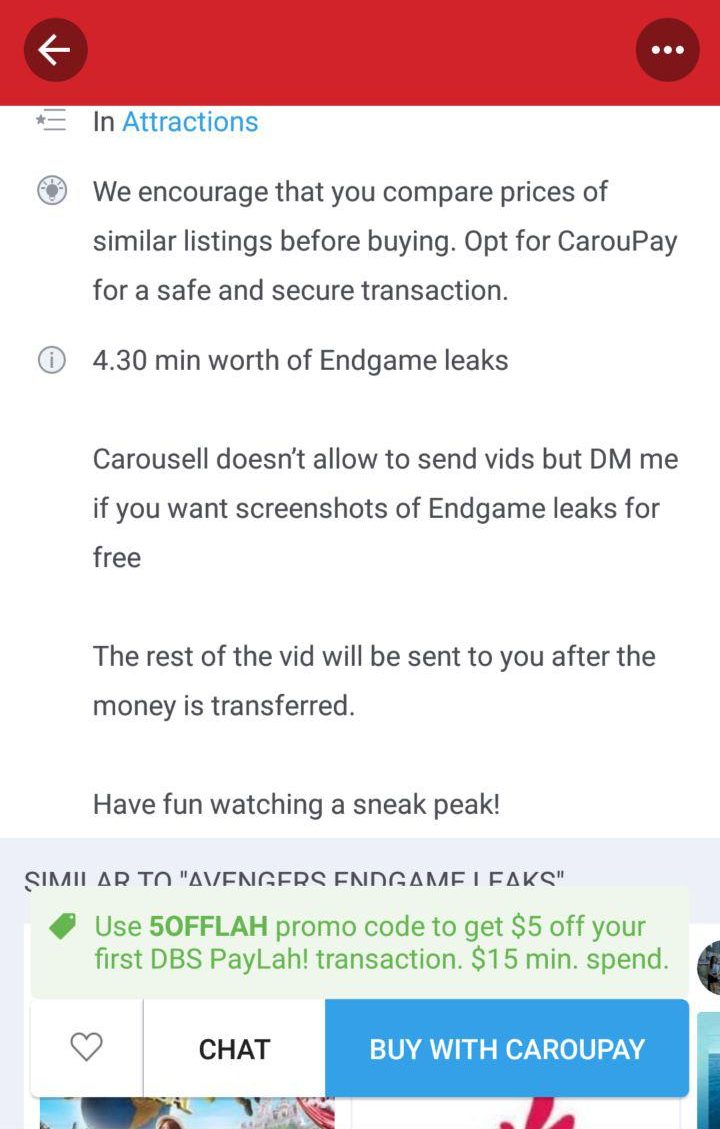The image features a complex array of icons and text. On the left, there is a red rectangle containing an arrow and a black circle pointing to the left. Adjacent to this on the right is a black circle with three dots inside it. Below that, the text "N Attractions" is displayed, with "N" in black and "Attractions" in blue.

Further down, there is an icon with a central black dot surrounded by lines, accompanied by the text: "We encourage you to compare prices of similar listings before buying. Opt for Carer Pay for a safe and secure transaction." Nearby, another icon resembling a clock is present, with the message: "430 minutes worth of in-game leaks. Carousel doesn't allow sending videos, but DM me if you want screenshots of in-game leaks for free. The rest of the video will be sent after money is transferred. Enjoy a sneak peek."

Towards the bottom, a gray rectangle carries the text "Similar to Avengers Endgame leaks," though its lower portion is obscured and hard to read. Above this gray rectangle, another gray bar states: "Use 50 FFLAH promo code and get $5 off your first DBS Paylah transaction. 15 minute spend."

Finally, at the bottom, a white rectangle houses three icons: a heart, a chat bubble, and a blue button with "Buy with Carer Pay" in white letters.